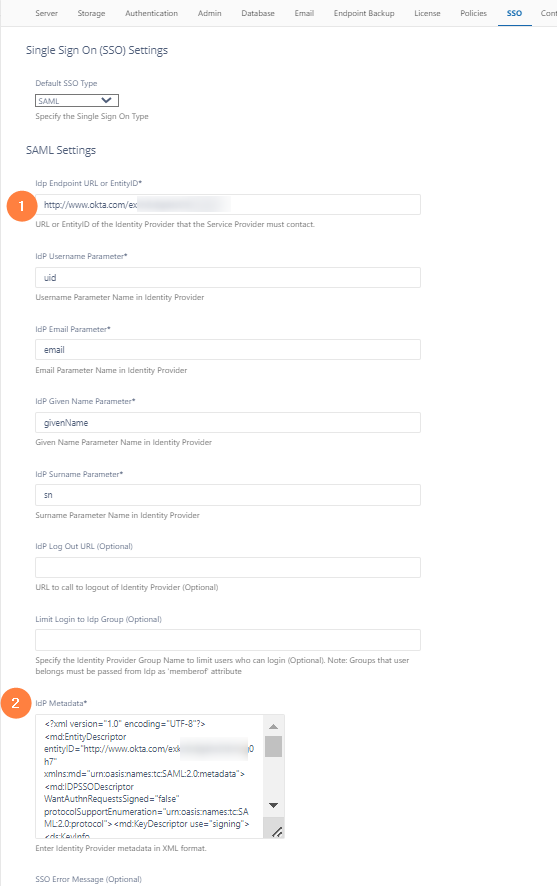This is a close-up shot of a highly detailed page, featuring a densely packed text that necessitated a substantial zoom for readability. At the top of the page, there is an evenly spaced menu bar, listing the following options from left to right: Server, Authentication, Actions, Database, Email, Desktop, License, Policies, SSO (highlighted in blue), and an additional Count option to the right. Directly beneath this menu bar, on the left side of the page, are the Single Sign-On (SSO) settings. This section first presents the "Default SSO Type" followed by a dropdown menu for selection. Below this, there are the SAML settings, clearly marked with a number "1" inside an orange circle on the left. Immediately following is another section indicated by a number "2" in an orange circle, detailing various settings or items listed within a distinguished sub-window. The entire layout is designed for navigation and configuration, catering to extensive customization and specific user requirements.